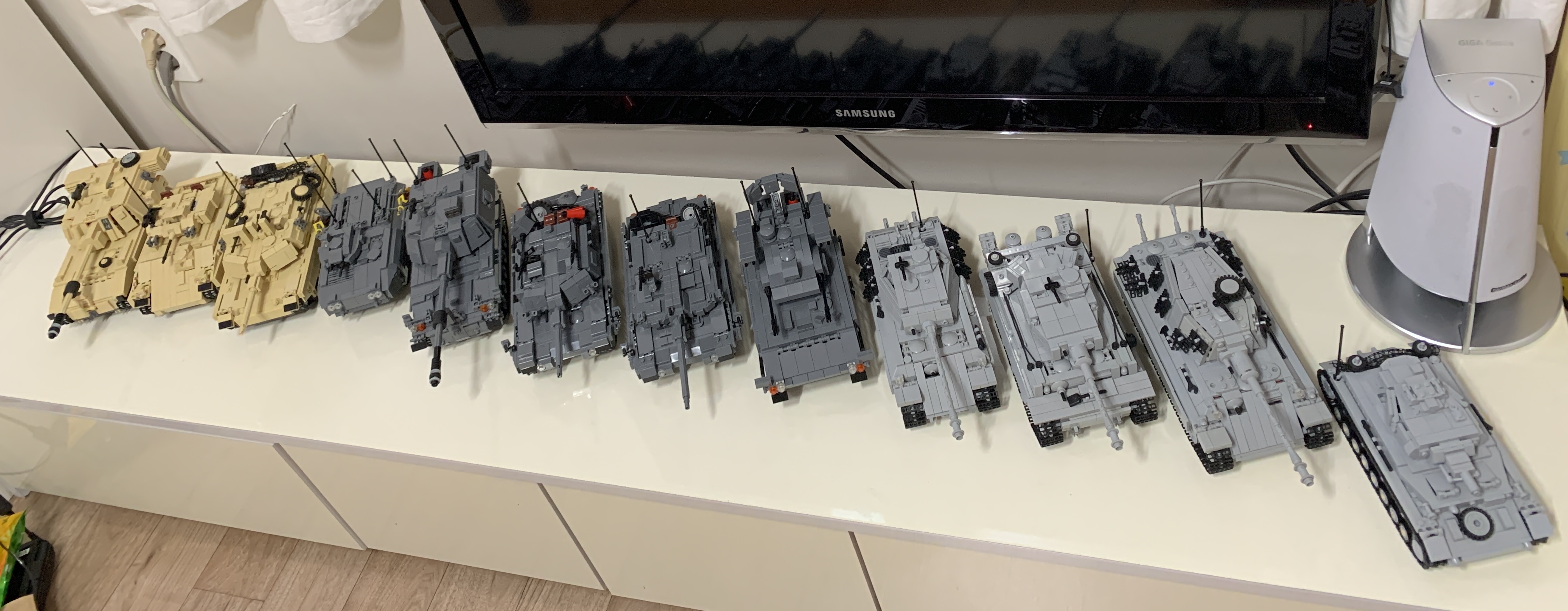This is a detailed photograph of a collection of twelve assembled Lego tanks, meticulously arranged on a white entertainment console beneath a flat-screen Samsung TV. To the left, three beige tanks sit side by side, followed by five dark gray tanks occupying the center of the shelf. On the rightmost side, four light gray tanks complete the lineup. Each tank is detailed with various black and red accessories, highlighting their different models and makes. The console itself is a sleek, white formica structure with drawers or cabinets below for storage. The visible floor surrounding the console is made of light tan wood panels. On the far right behind the light gray tanks, there is an unidentified white device, possibly a humidifier or a gaming console, enhancing the modern entertainment setup.